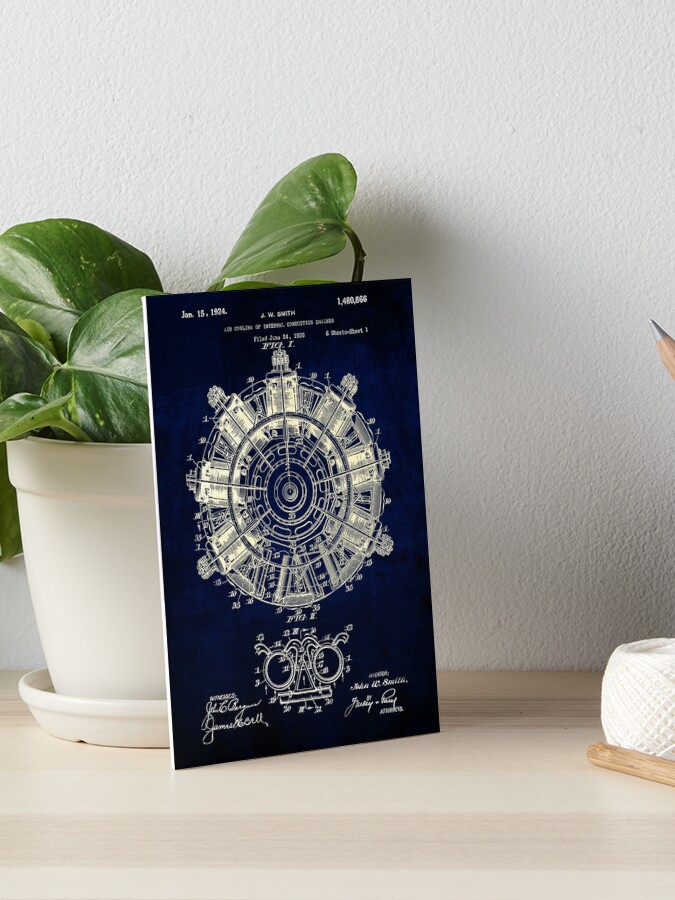The image depicts a small, dark navy booklet or poster leaning against both a white wall and an off-white, cream-colored indoor flower pot with green leafy plants. The backdrop also includes a very light, almost white, beige wooden floor. In the center of the booklet or poster, there is a circular emblem resembling a compass with prongs around it and what appears to be similar to eyeglasses towards the bottom. The booklet is adorned with various pieces of text, though most are unreadable; however, notable elements include the date "January 15, 1924," the name "J.W. Smith," and the label "figure one," along with more cursive text at the bottom that is too blurry to discern.